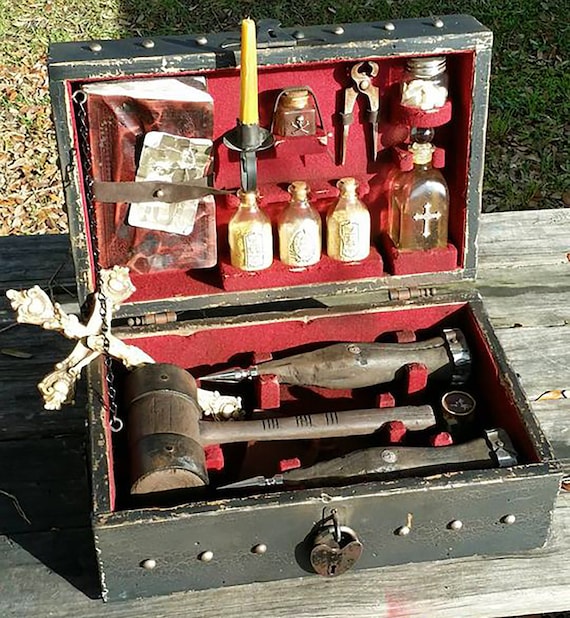This detailed photo captures a vintage-looking wooden toolbox, which seems to be set on a rustic picnic table outdoors, evident from the grass visible in the background. The chest's exterior, though painted black, is chipped and worn, giving it an antique feel. 

A heart-shaped padlock secures the front of the chest. The box is open, revealing a red velvet lining inside both the top and bottom compartments. The bottom half features an assortment of old tools and relics. Dominating the left side is a large wooden mallet, spreading horizontally with its head on the left and handle pointing to the right. There are also two pointed wooden stakes, each capped with silver tips, arranged near the mallet. Intriguingly, a golden ornate cross rests at the bottom, partially protruding out, adding to the mystical allure.

The upper section of the toolbox is equally captivating. On the left side, a disheveled book is securely strapped in place. To its right, several old bottles are neatly arranged, many adorned with crosses, their contents undetermined but suggestive of mysterious potions or remedies. Additionally, there's a yellow candle in a black holder, a set of pliers, and what appears to be a small, rounded object. The presence of a small box featuring a skull and crossbones further enhances the impression of this being a specialized kit, possibly intended for combating supernatural entities like vampires.

The meticulous assembly of these eclectic items, combined with the red velvet interior and the heart-shaped padlock, underscores a narrative steeped in history, mystery, and perhaps even the fantastical pursuit of vampire hunting.